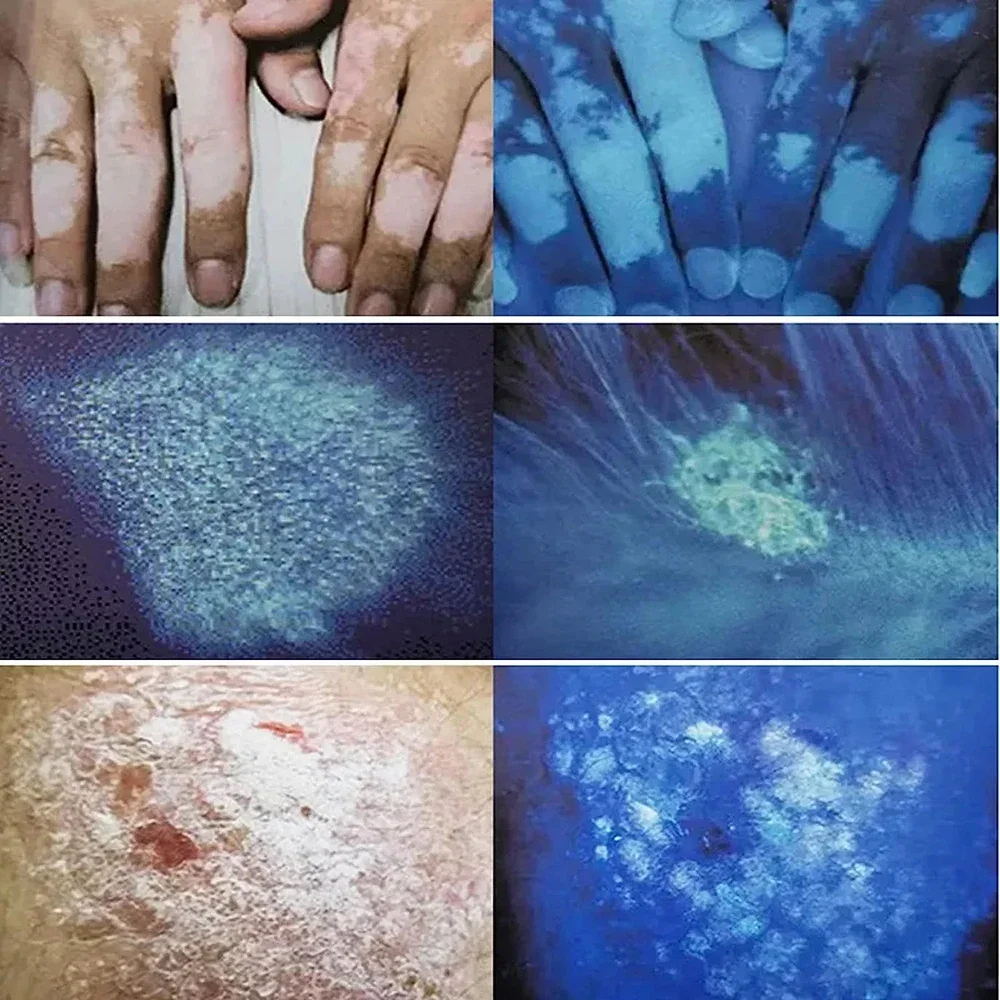This series of six photographs illustrates various skin conditions, captured under both normal and blacklight conditions in a grid of two across and three down. The top left image shows fingers affected by vitiligo, with skin partially beige-brown and partially pink. The top right image captures the same fingers under blacklight, highlighting patches of deep blue and light blue. 

The second row features two images of skin under blacklight. The left photo displays a blue-tinted area with numerous white dots, suggesting a spray-painted effect, related to a skin condition that appears to glow under the light. The right image in this row looks like a wave with large dark blue and purple patches, and a dense spiderweb-like white splotchy center, potentially indicating another skin irregularity.

The bottom row contains images of skin conditions that have a different texture and composition. On the left, a color photo captures a view resembling a salt lake with beige areas, red rocks, and spread white salt, likely indicative of dry skin conditions such as psoriasis or eczema. The corresponding bottom right image shows the same skin under blacklight, resembling a deep blue ocean scene with white rocks scattered in the center.